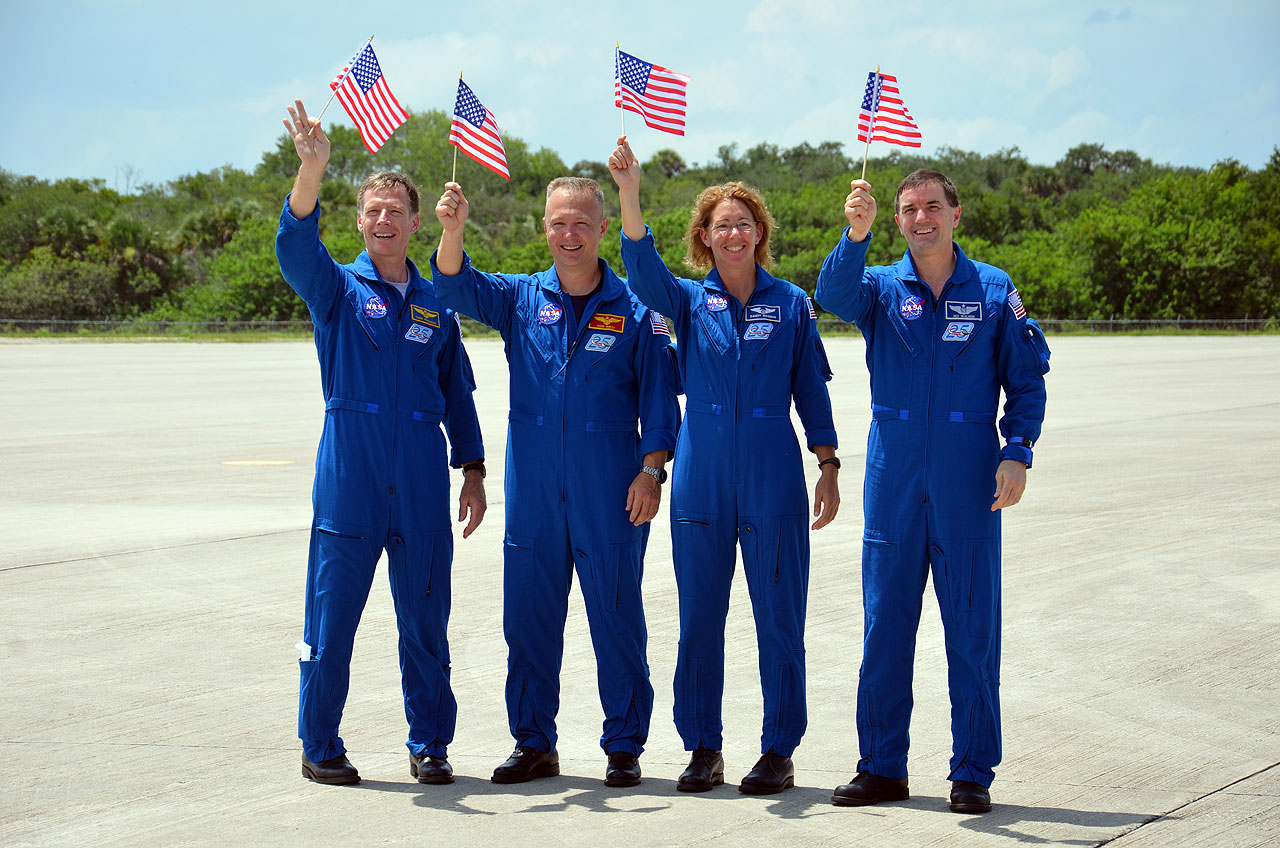In this photo, we see four NASA astronauts, consisting of three men and one woman, standing in a row on what appears to be an airfield at Cape Canaveral. They are all dressed in blue uniforms, each adorned with patches and pocket sleeves. The astronauts are smiling broadly and holding small wooden poles with American flags in their right hands, while their left hands rest at their sides. 

The astronaut on the far left has short brown hair and no facial hair. Next to him is a man with a buzz cut and gray hair, possibly sporting Navy wings on his lapel. The woman standing third in line has short reddish-orange hair and glasses. The man on the far right has short brown hair and no facial hair, and he may be wearing Marine Corps wings. The rest appear to have Air Force wings. They are all Caucasian and wear black shoes.

The background features a brilliant blue sky with minimal cloud coverage, verdant trees, and the asphalt ground, hinting at a sunny day. Shadows suggest early afternoon light, casting a gentle illumination over the scene. This image might depict the crew from the last shuttle mission in 2011.